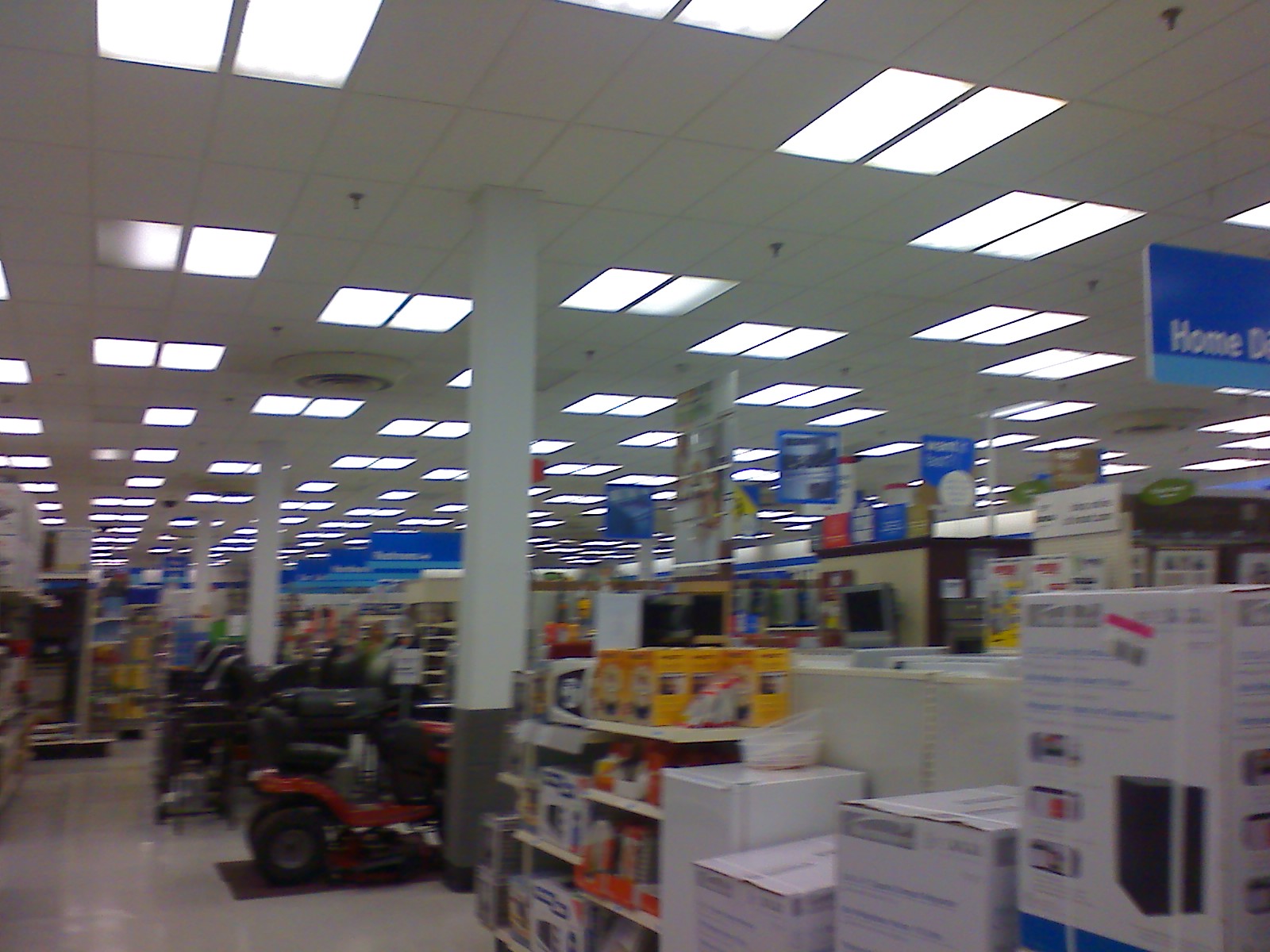A blurry, low-quality image taken inside a supermarket captures a chaotic scene of shelves stocked with various products. Numerous refrigerators line the aisles, and a surprising sight of a motorcycle stands amidst the retail setting. There are several signs in the shot, with the closest one partially readable, displaying "Home D." The overall lack of focus and clarity makes it difficult to discern specific details, contributing to the image’s overall indistinct and disordered appearance.